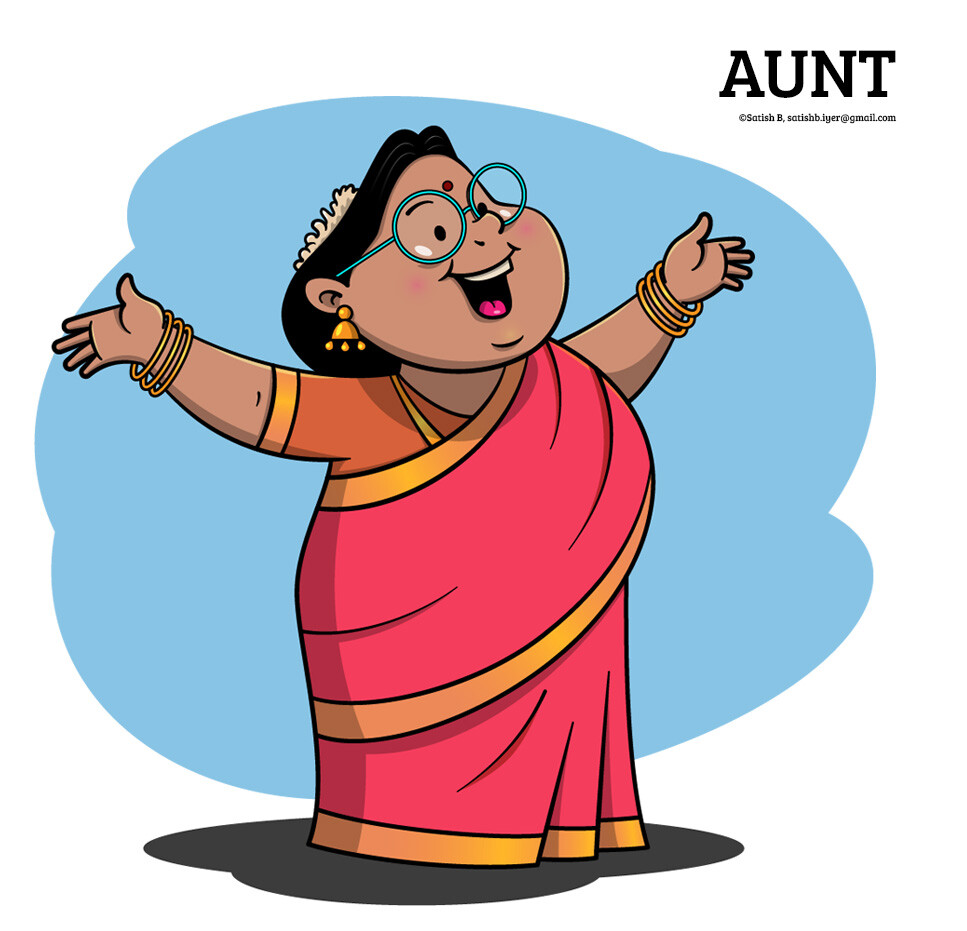This image features a vibrant, cartoon-style 3D artwork of an exuberant Indian woman with a joyful expression, arms spread wide. At the top right corner, the word "ant" is written in black, accompanied by a copyright note crediting "Satish B" alongside an email address. The woman, portrayed with a round and chubby figure, is surrounded by a blue background that acts as a watermark.

She has brown skin, rosy red cheeks, and a bright pink tongue visible between her smiling white teeth. Her large, round, teal-colored glasses stand out prominently. She has black hair, and on her right ear, she's adorned with yellow, bell-shaped earrings that feature three small golden circles at the bottom. The woman's attire consists of a reddish-pink robe with golden trim, wrapped around her chest and draped down like a dress, along with a short-sleeved orange shirt featuring golden trim near her elbow. On her wrists, she wears three golden looped bracelets on both arms. This detailed and colorful depiction captures the essence of cultural attire and joyous spirit.